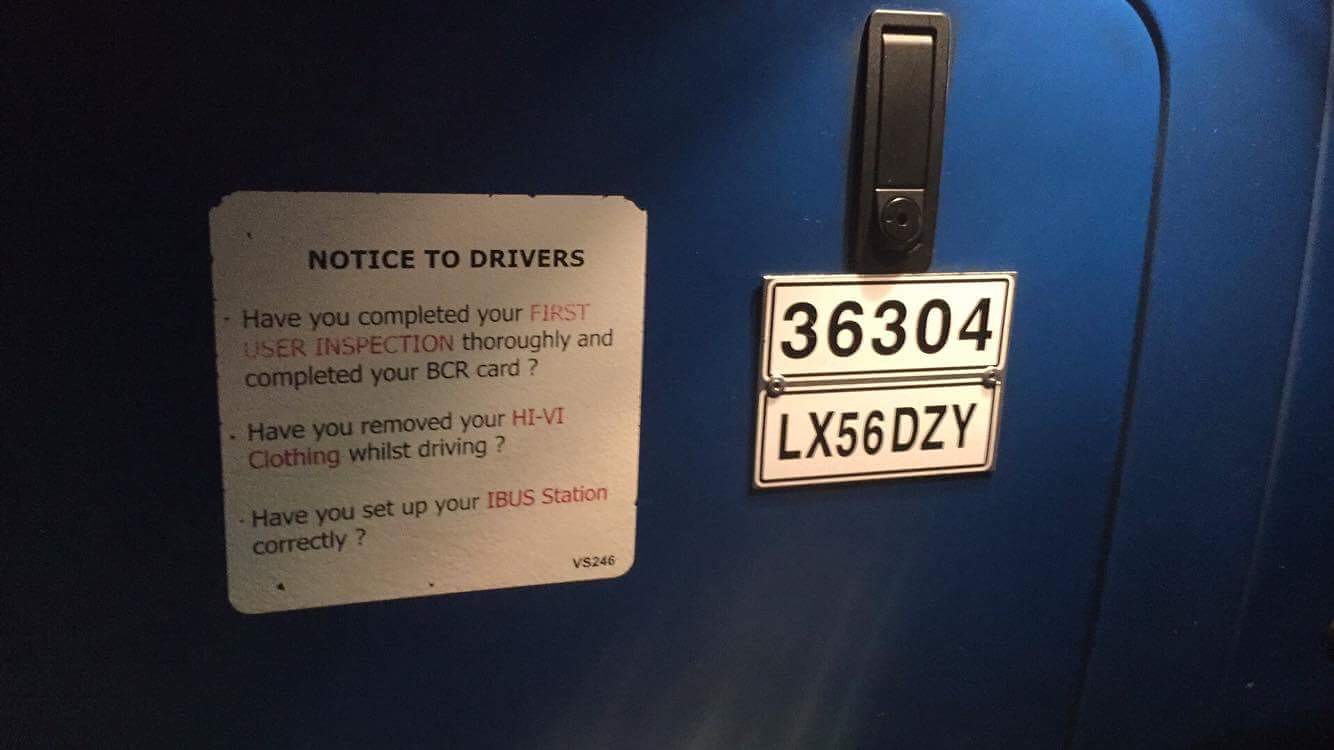The image depicts a blue door featuring important notices for drivers. 

On the left side, there is a white square plaque with black and red text titled "Notice to Drivers." The plaque lists three bullet points:
1. Have you completed your first user inspection thoroughly and completed your BCR card?
2. Have you removed your Hi-Vis clothing whilst driving?
3. Have you set up your iBus station correctly?

Additionally, at the bottom of this notice is the code "VS246."

On the right side, two white tags, resembling license plates with black borders, display alphanumeric codes. The first tag reads "36304" and the second one "LX56DZY." Above these tags, there is a small lock with a push button and key mechanism.